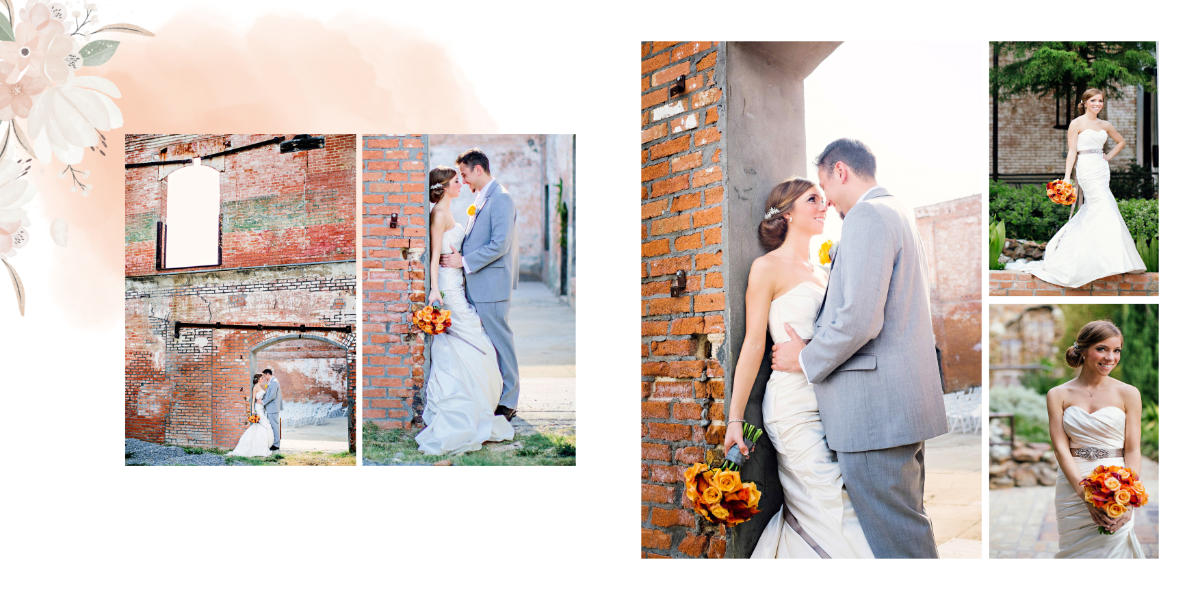The image appears to be a wedding card featuring a carefully curated arrangement of five main elements. Dominating the upper left-hand corner is a delicate watercolor illustration with light orange clouds and a flower consisting of white and green leaves along with a light orange head. The card includes photographs set against a generous white space backdrop, lending an air of elegance and simplicity.

Four of the photos capture the intimate moments of a couple's wedding day. The bride is dressed in a long white gown and holds a bouquet of orange and yellow flowers, which are reminiscent of fall colors, possibly roses. Her dark hair contrasts beautifully with her attire. The groom is in a gray or blue suit, complemented by a yellow flower in his lapel.

Two pictures feature the couple together; one of them is set against a rustic brick building that exudes old-world charm, characterized by varied brick tones. Another photo captures the couple posed intimately near a doorway. Additionally, there are two solo pictures of the bride in different poses, showcasing her bouquet and bringing further attention to her elegant appearance.